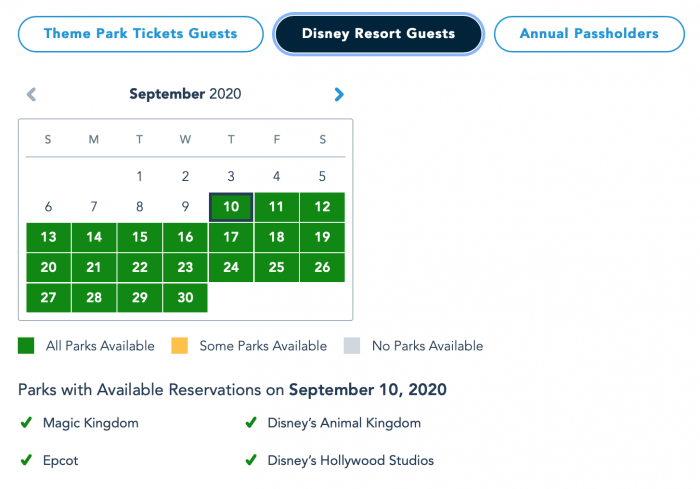The image depicts a detailed calendar interface prominently featuring the month of September 2020. Positioned to the left is a calendar header with "September" in bold lettering and "2020" in regular font. A disabled light gray left arrow and an active blue right arrow flank this header. Below the month and year, the days of the week, abbreviated as S, M, T, W, T, F, S and spaced out to signify Sunday through Saturday, are clearly labeled.

The calendar itself displays the dates from 1 to 30. Notably, the dates from the 10th to the 30th are highlighted within green boxes, with the 10th date box further outlined in a dark gray or black border.

At the bottom of the calendar, a legend explains the color coding: green signifies "all parks available," yellow indicates "some parks available," and gray denotes "no parks available." A bold heading reads, "Parks with available reservations on September 10th, 2020," followed by a green check mark. Listed beneath are the parks with available reservations: Magic Kingdom, Epcot, Disney's Animal Kingdom, and Disney's Hollywood Studios.

The top left of the interface features a blue-bordered, elongated oval containing the text "Theme Park Ticket Guests" in blue writing. Adjacent to it, another similar oval shape with a dark blue background and white lettering reads "Disney Resort Guests," indicating it is selected. Further right, another blue-bordered oval states "Annual Pass Holders."

The calendar itself is rectangular, outlined in light gray. Below the days of the week, a light gray border line runs horizontally.

Finally, each headline in the bulleted list on the interface's left is preceded by a small dark green check mark, adding a cohesive visual element to the design.